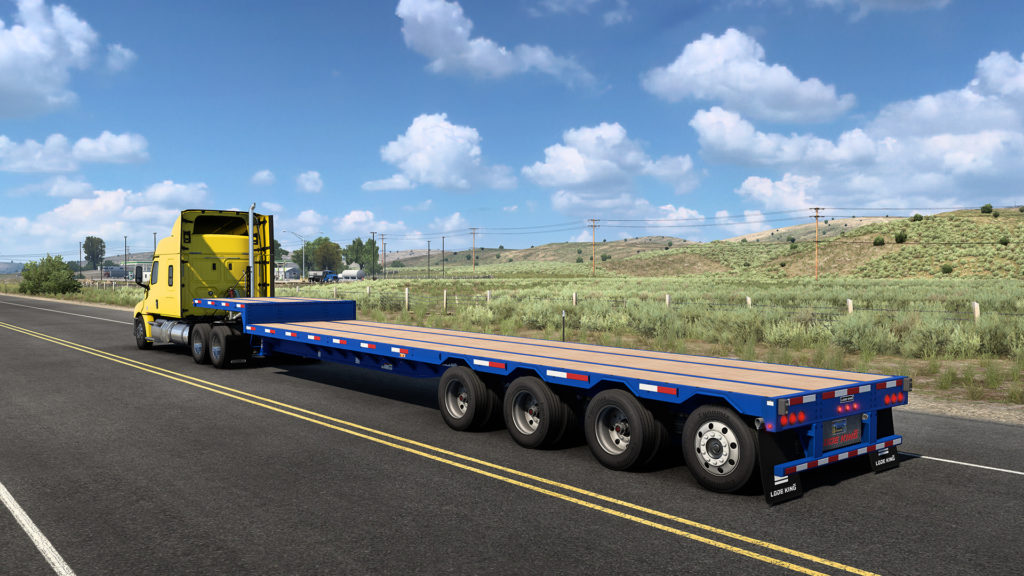The image depicts a long, stationary 14-wheeler tractor trailer parked on a newly paved, dark gray highway adorned with yellow center lines. The front of the truck is distinctly yellow with silver accents, while the flatbed at the back features blue sides and back with a light beige top. Nestled in a serene landscape, the scene includes a grassy hill beside the road, though the grass appears spotty and not very healthy, with a soft light green hue. White posts with wire, a couple of trees, and power lines are visible in the background. Above, a blue sky filled with fluffy white clouds completes the picturesque setting.